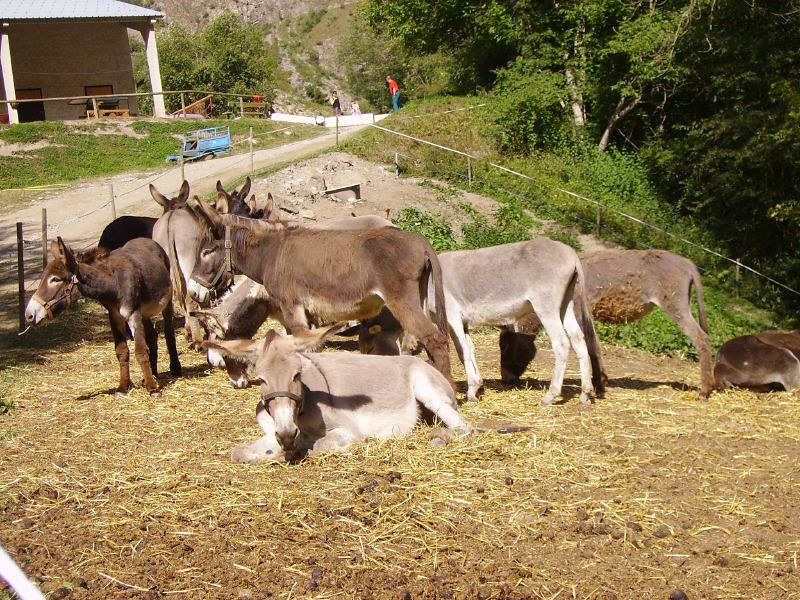The photograph captures a serene outdoor scene on a large farm. Dominated by a small herd of donkeys, both standing and lying on a hay-strewn, light tan ground, the image includes around ten donkeys in total, displaying shades of light grey and light brown. The donkey in the foreground, light grey in color, is lying down and almost looking directly at the camera, while the others are positioned facing various directions, with a couple eating from the ground. The farm is enclosed with a white roped fence, and in the backdrop, lush greenery comprising trees and bushes fills the scene. 

Further back, a dirt road divides two grass fields, with a blue wheelbarrow or rolling structure near the fence. Towards the road, we see three indistinct figures - a man in a red shirt, a woman, and possibly a child, standing together, their facial features obscured by the distance. Additionally, part of the landscape includes a large, grey building or barn, perhaps still under construction, situated towards the top right of the image. The overall atmosphere is a peaceful depiction of rural farm life, with various elements harmoniously coexisting.